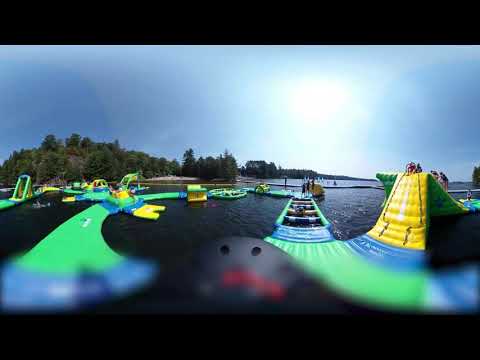The image is an outdoor daylight photograph of an expansive, dark-blue body of water taken from the water looking towards the shore. The photo is bounded at the top and bottom by black bars, giving it a widescreen, possibly 360-degree image feel that has been flattened for two-dimensional viewing. On the water's glittering surface are numerous inflatable structures and interconnected play areas, characterized by ramps, slides, paths, and climbing areas in vibrant colors of blue, yellow, green, and white. Prominently on the right side of the image, several people, including small children, are seen climbing a yellow slide ramp. To the left, there is a curving green path leading to further inflatable attractions that meet in the middle distance. The shore in the background shows a hilly landmass lush with dark green trees and bushes, and there is a visible building in the far distance. The sky overhead is a deep, cloudless blue, dominated by bright sunlight illuminating the playful, floating amusement park.